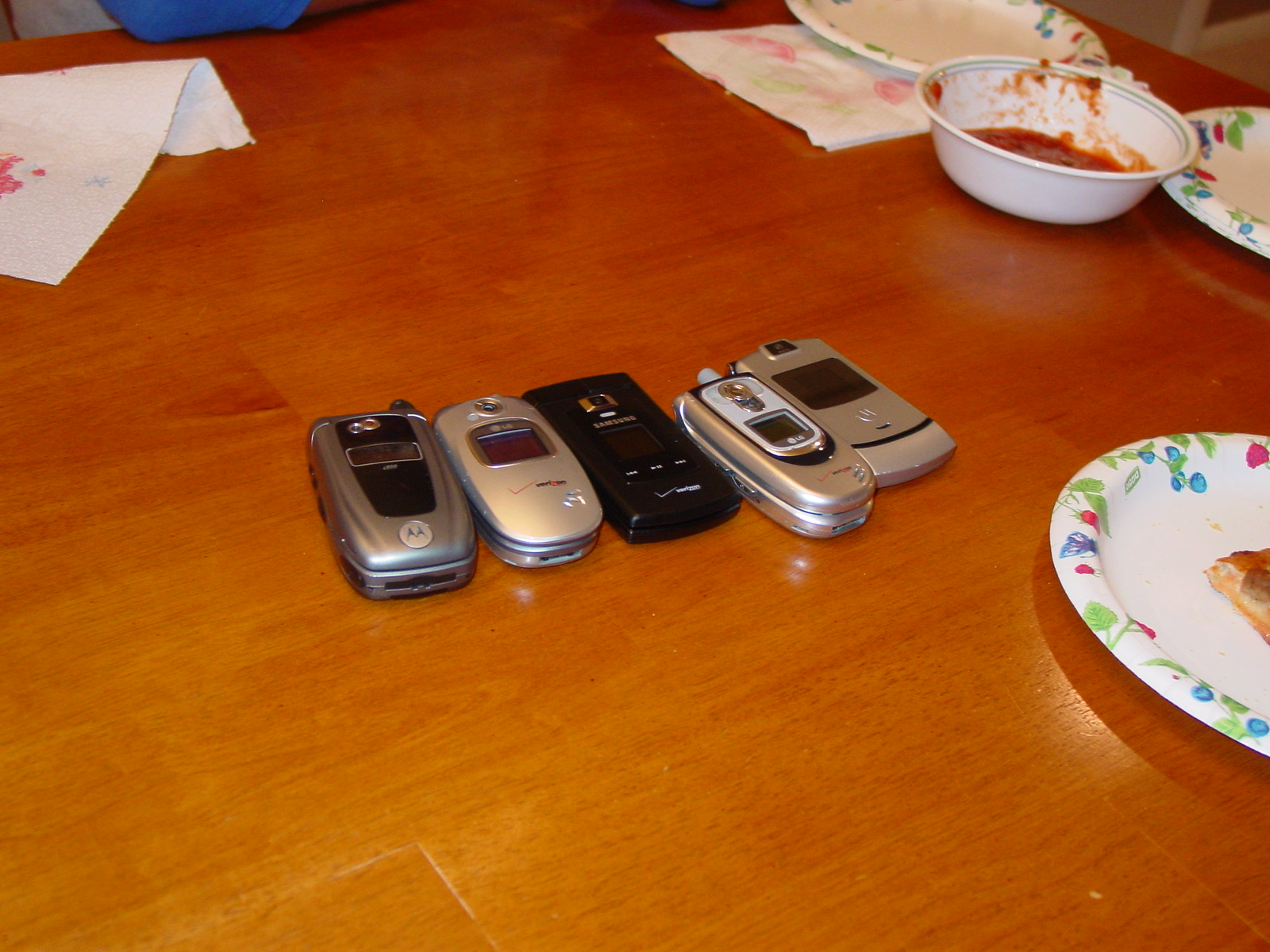In this detailed photograph, a varnished reddish-brown wooden table dominates the scene. At the center of the table, five clamshell flip phones are carefully lined up, suggesting perhaps a personal collection of older mobile phones. Most of these phones are silver, with logos indicating brands like Motorola and Verizon, while one phone in the middle stands out in a black color. Each phone features a small LCD display and a camera on the front.

Surrounding the phones are several white paper plates adorned with pastel-colored edges in shades of green, blue, and pink. One plate rests on a white serviette with light pink blotches, possibly from food. A small white bowl containing a reddish sauce sits on the table, and additional serviettes are visible in the top left corner of the image. The overall arrangement gives the impression of a recently finished meal with remnants of food and dining utensils scattered across the table.